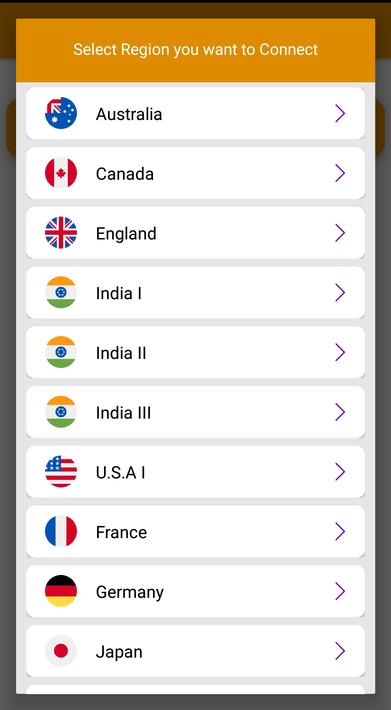The image depicts a printout of a regional listing interface. At the top, there is an orange background bar with the text "Select Region You Want to Connect" spanning from left to right. Below this header, there is a series of rows, each representing a different country. 

- The first row lists "Australia" accompanied by its logo and a clickable symbol to the right.
- The second row lists "Canada," also with its logo and a clickable icon to the right.
- The third row lists "England" with its logo and a clickable icon to the right.
- The fourth row lists "India One" with its logo and a clickable icon to the right.
- The fifth row lists "India Two" with its logo and a clickable icon to the right.
- The sixth row lists "India Three" with its logo and a clickable icon to the right.
- The seventh row lists "USA One" with its logo and a clickable icon to the right.
- The eighth row lists "France" with its logo and a clickable icon to the right.
- The ninth row lists "Germany" with its logo and a clickable icon to the right.
- The tenth row lists "Japan" with its logo and a clickable icon to the right.

None of the countries in the list have been selected yet.